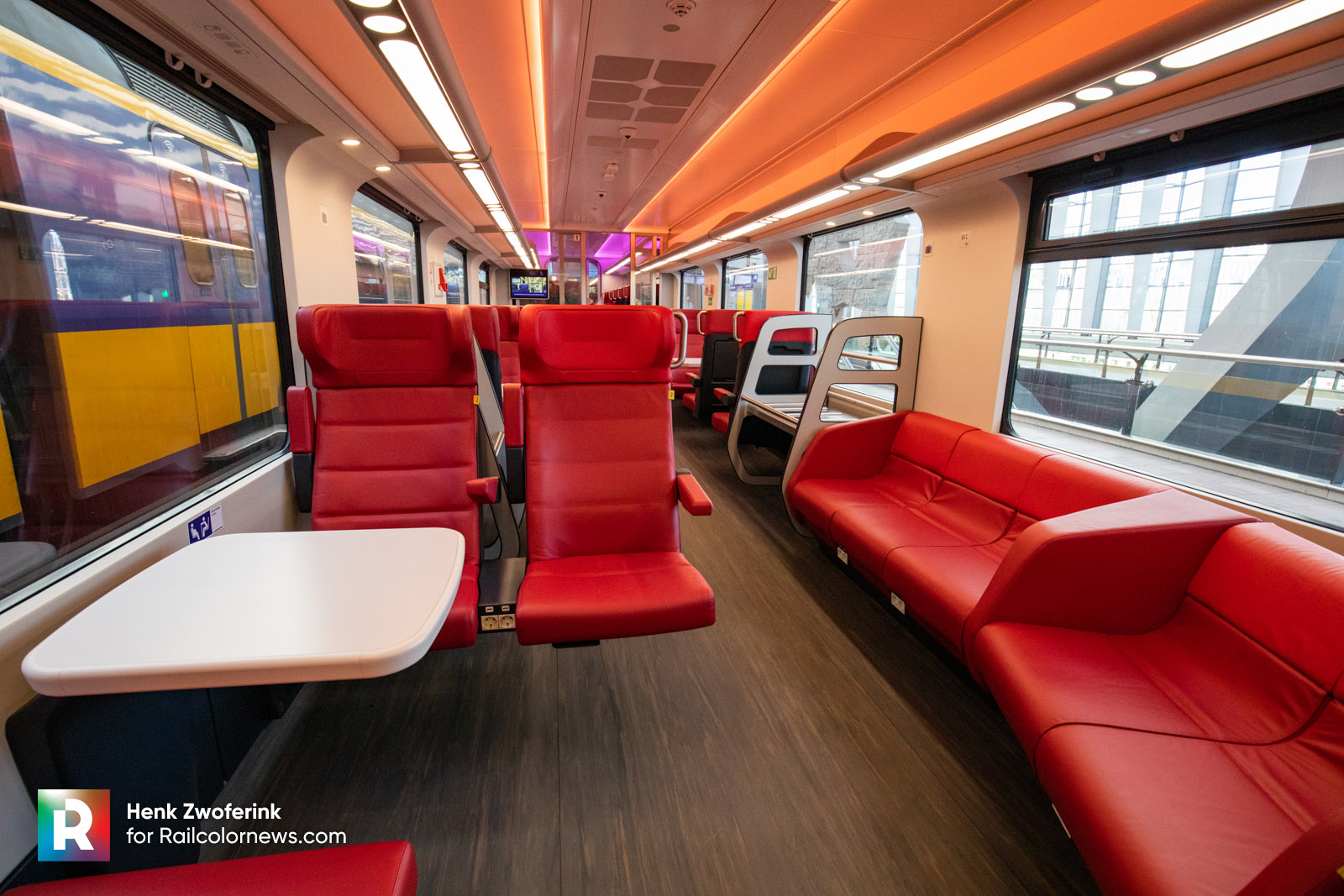The image depicts the futuristic and spacious interior of a modern train or subway car stationed at a platform. The car is brightly lit with mood-enhancing ceiling lights, featuring an orangey glow and purple accents. To the left, large windows offer a view of another train, while windows on the right reveal buildings and railings. The interior boasts a mix of floating and bench-style seating, all upholstered in vibrant red leather. The floating seats on the left side come with armrests and small white tables perfect for placing a laptop or other items, while red leather bench seats are situated on the right side of the car. Further back, more seating options and additional railings can be seen. In the bottom left corner of the image, a square logo with rainbow colors surrounding a bold "R" is present, alongside text that reads "Hank Zwofaring for railcolornews.com."